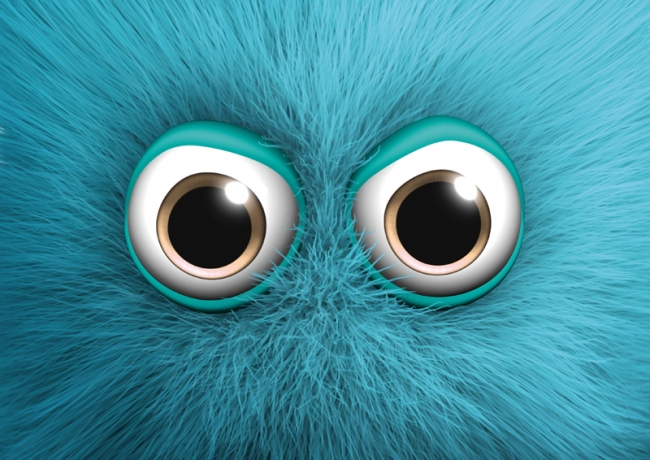The image depicts a close-up of a computer-generated, blue furry creature, focusing prominently on its eyes. Surrounded by teal, 3D-shaded eyelids, the eyes themselves appear large and slightly rounded. The main portion of each eye is a very light grey, almost off-white. Encircling the heavily dilated black pupils is a brown iris, transitioning to a lighter brown at the bottom. There is a noticeable reflection of light in the top right corner of each pupil. The creature's fur, composed of long strands resembling hair, is a vibrant turquoise blue. The entire composition is slightly rectangular and framed horizontally, with shading details adding a realistic texture to the fur. The image emphasizes the creature's gaze, devoid of any visible mouth, enhancing the eerie yet captivating focus on its expressive eyes.